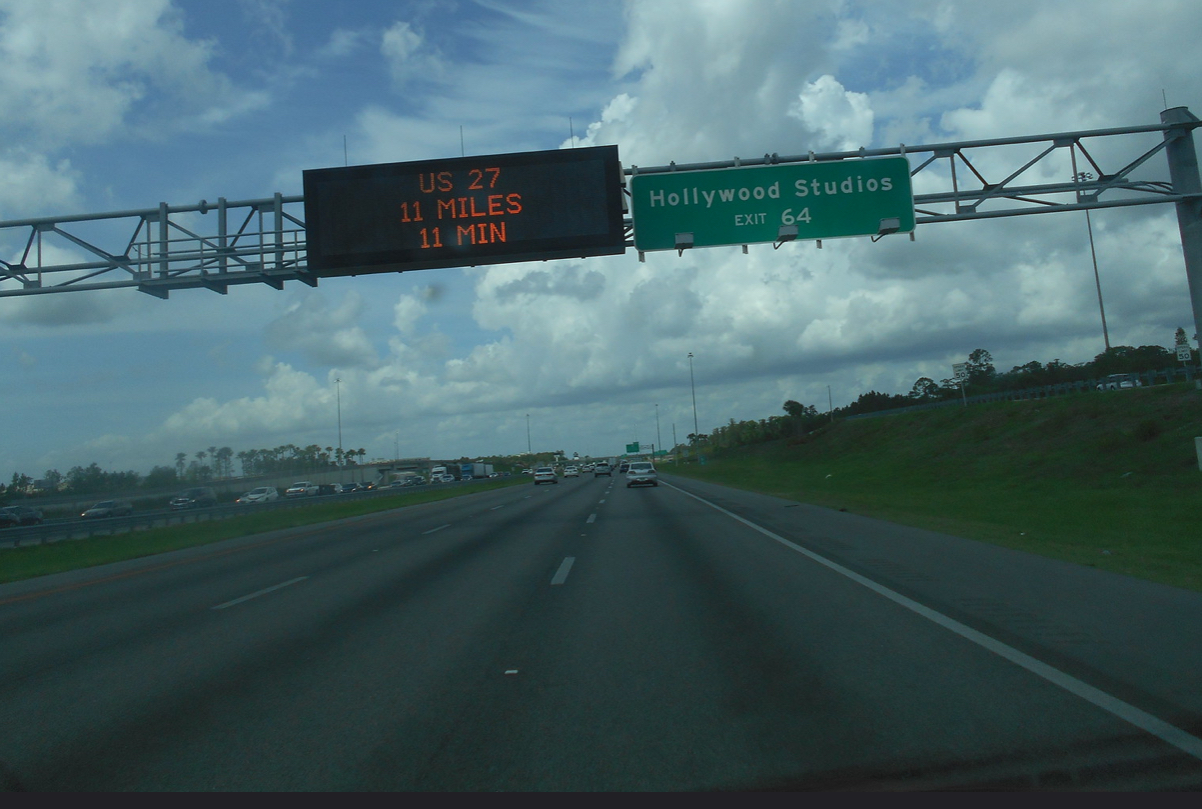The image depicts a three-lane highway with an overhead metal structure holding several signs. One of the signs is green with white lettering, indicating an exit for Hollywood Studios, labeled as Exit 64. Adjacent to this, there is an electronic sign with black edging and background, displaying the message "U.S. 27, 11 miles, 11 minutes." The median separating the lanes is composed of dark gray tar, while the sides of the highway feature overgrown green grass that slopes upwards into a hill.

To the right, a car is seen descending onto the freeway, merging from an exit. Ahead on the highway, a white car is visible along with a few other vehicles. White dotted lines mark the lanes, and a green grassy median, bordered by a guardrail, separates the opposite-flowing traffic. On the opposite side, more cars are observed traveling in the other direction. The sky overhead is light blue, filled with numerous puffy white clouds, covering much of the skyline.